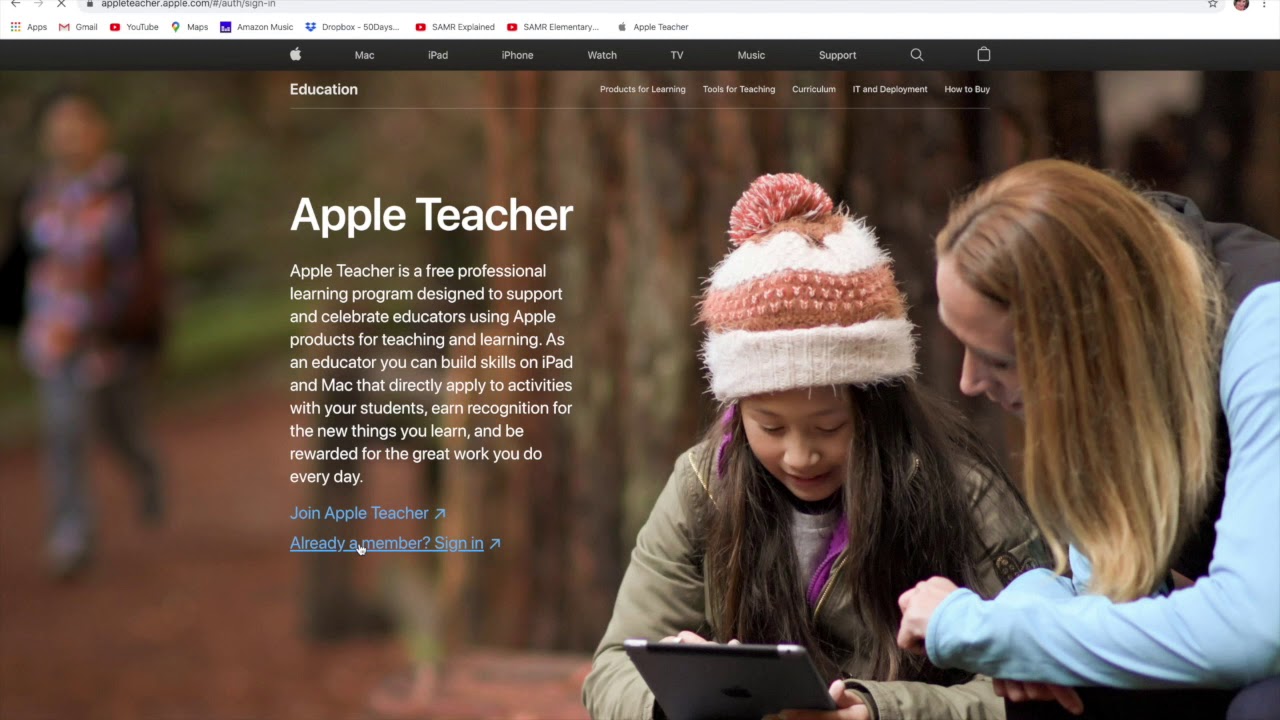This image captures the Apple website's education section, where a user has navigated to a specific panel focused on educational resources. The central visual features a child engaged with an iPad while being assisted by a teacher, depicting an interactive learning experience. To the left of this image, there's informative text under the heading "Apple Teacher," which is prominently displayed in white uppercase letters. The accompanying paragraph describes "Apple Teacher" as a complimentary professional learning program dedicated to supporting and celebrating educators who incorporate Apple products into their teaching practices.

Above this main section, a series of navigation headings is displayed, including options such as "Education," "Products for Learning," "Tools for Teaching," "Curriculum," "IT and Deployment," and "How to Buy." Further up, a grey navigation bar can be seen featuring additional headings. On the far left, the iconic Apple logo is visibly placed, followed by links to "Mac," "iPad," "iPhone," "Watch," "TV," "Music," and "Support," as well as a search icon. A final, unclear icon, resembling a clipboard, is also included in this top navigation bar. The overall layout emphasizes Apple's commitment to integrating technology into educational environments.